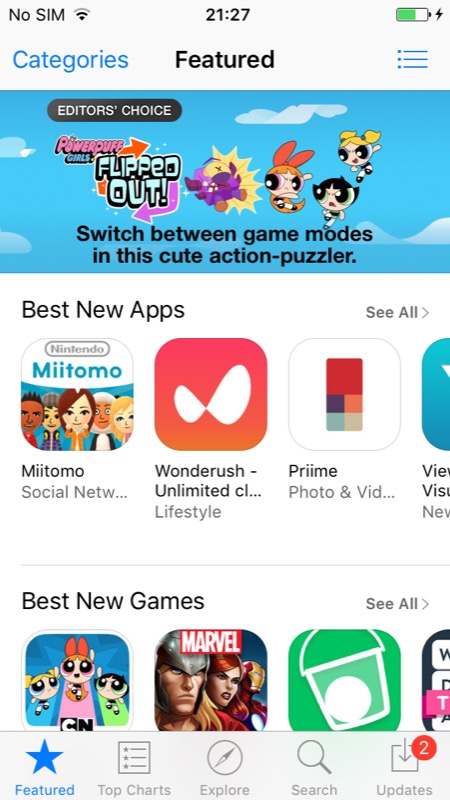The image displays a screenshot of a web page, likely from a mobile app store. On the left-hand side, the status bar indicates "No SIM" and the time reads 21:27. A green bar at the top right displays the battery life, which is at half capacity.

The main content area contains several sections. To the left, there is a navigation menu with the item "Categories" listed prominently. Below this, the word "Features" is visible. On the right side of the screen, three blue horizontal lines act as a menu button.

Central to the image, there is a prominent feature section showcasing "The Powerpuff Girls" flying with a caption "Flipped Out." Below, a second image depicts a purple character labeled as "Editor's Choice" with a description encouraging users to switch between game modes in a "cute action puzzler."

Further down, a section titled "Best New Apps" displays several apps including "Miitomo," "Wonder Brush Unlimited," and "Prime," along with a partially cut-off app. Additionally, a "Best New Games" section features "The Powerpuff Girls," "Marvel," and what appears to be an image of a paint bucket, possibly representing a painting app or game, among others that are partially obscured.

At the bottom, navigation options include "Featured," "Top Charts," "Explore," "Search," and "Updates." Next to "Updates," a red circle with the number two indicates two pending updates.